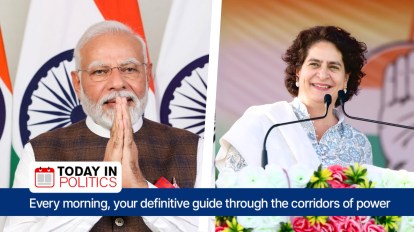The detailed caption for the image would be:

"This photograph appears to be a screenshot from a television news program, labeled 'Today in Politics' with the tagline, 'Every Morning, Your Definitive Guide Through the Corridors of Power' written in blue text at the bottom. On the left side, there is an older man with gray hair, glasses, gray eyebrows, and a full gray beard and mustache. He is wearing a white collared shirt with a brown vest over it and stands in a stance with his hands clasped together up to his face, in a prayer position. Behind him are flags that are white with orange and blue. On the right side, there is a woman smiling in front of two small microphones. She has short, dark hair and is wearing earrings and a blue collared shirt with a white sari draped over one shoulder. Her floral attire features colorful patterns. In the background, there is a flag with shades of green, white, and yellow and symbols below it."